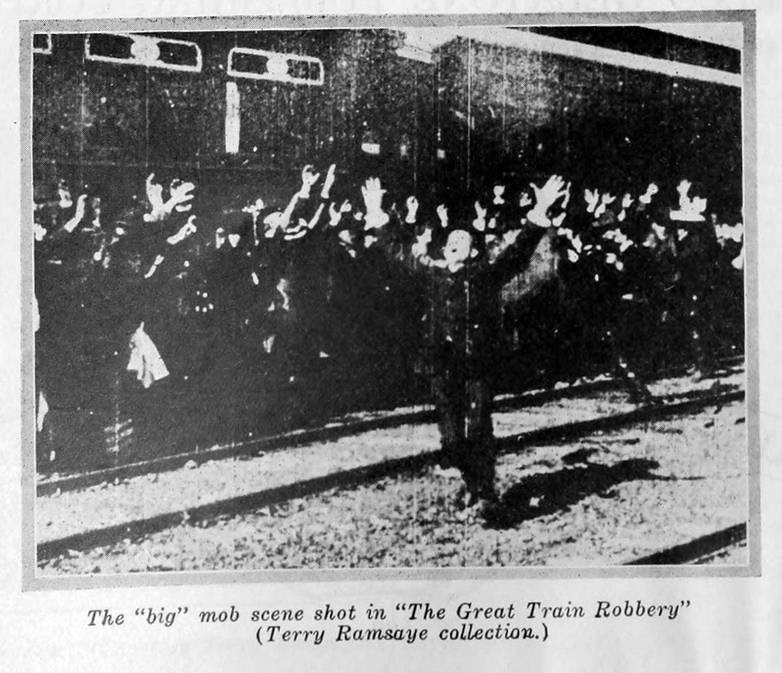This grainy, black-and-white photograph, evidently from the Terry Ramsey collection, captures a dramatic moment described as "the big mob scene shot in The Great Train Robbery." The image, although of poor quality, depicts a large group of people, all with their hands raised towards the sky, palms out. They appear to be shouting or yelling, creating a chaotic atmosphere. At the center of the group, yet set apart, is a man with his hands also raised and mouth agape, suggesting he is leading or reacting strongly. The scene unfolds next to train tracks, with a train barely discernible in the background due to the image's poor quality. Despite the indistinct background, the collective gesture of the mob and the solitary figure at the front are the photo's focal points, poignantly conveying a moment of tension or urgency.